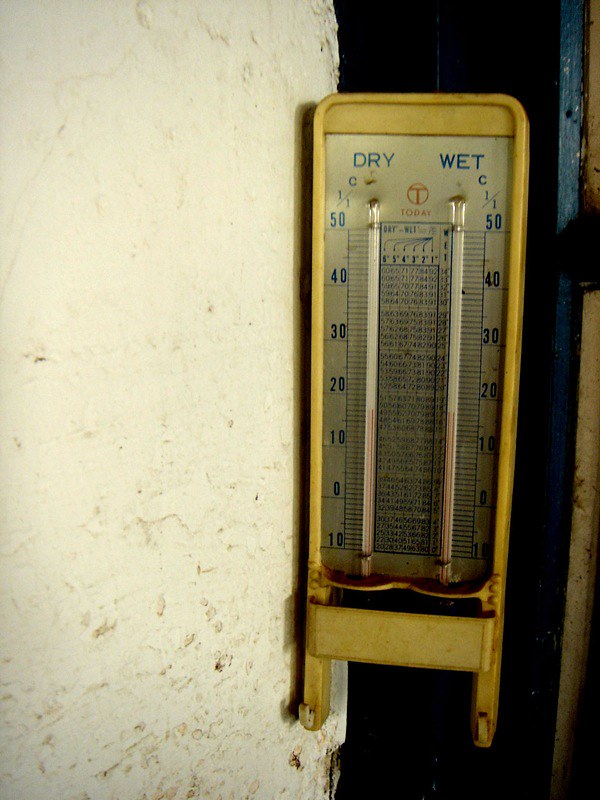This image depicts a dual thermometer designed to measure both dry and wet temperatures, mounted on a yellow metallic base. The base, shaped somewhat like a sled with two small legs at the bottom, is affixed to the side of a grimy white wall. The wall itself bears numerous scratches, scuff marks, and scattered brown stains, giving it a distinctly weathered appearance.

Each of the two long, slender thermometers are positioned side by side, with visible red liquid rising from the base, indicating temperature readings. The temperature scale on the thermometer ranges from -10 to 50 degrees, with both thermometers displaying approximately 17 degrees. Inside the thermometer casing, a chart is visible featuring numerous blue lines and numbers that appear unreadable in this image.

At the top of the thermometer, where the two sides end, the left side is labeled "Dry" in blue text, while the right side is labeled "Wet." Between the two labels, an orange circle with a 'T' inside is present above the word "Today," which is written in capital letters and also colored orange.